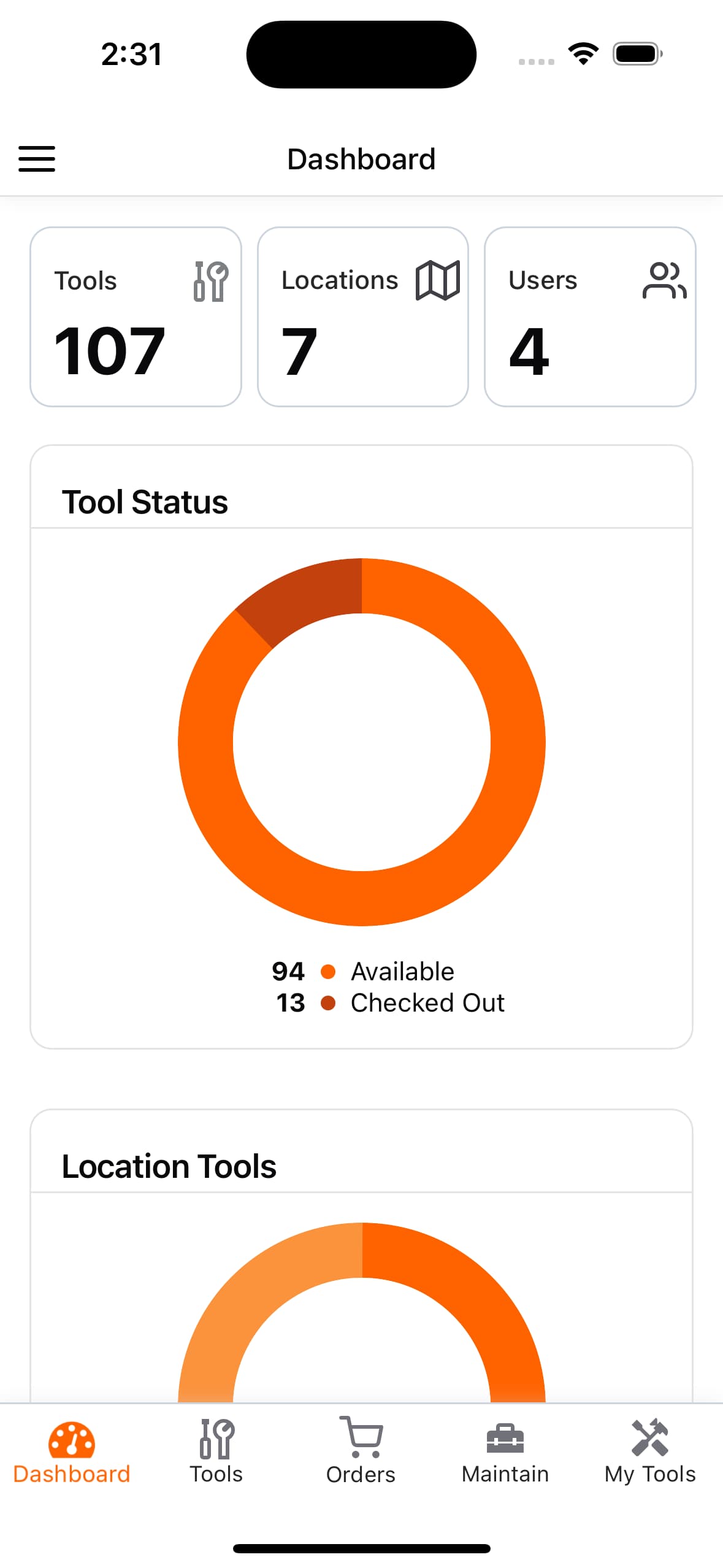This image is a detailed screenshot from a cell phone displaying a dashboard interface. At the top of the screenshot, the title reads "231 Dashboard." Below the title, there are several sections with corresponding icons: "Tools, 107" is accompanied by an icon of a wrench and a screwdriver, "Locations, 7" is paired with a folded map icon, and "Users, 4" is represented by an icon of a person with another person positioned slightly behind them.

Under these sections, there's a "Tool Status" indicator featuring a prominent circular graphic. This graphic is divided into two segments: a large light orange section indicating "94 available" tools, and a smaller dark orange segment showing "13 checked out" tools. The circle is slightly truncated at the bottom edge.

At the bottom of the screenshot, there is a navigation bar with several options. Each option is represented by both text and icons: "Dashboard" is highlighted in orange and marked with an icon of an orange speedometer with white details, "Tools" has the wrench and screwdriver icon, "Orders" is illustrated with a shopping cart icon, "Maintain" is shown with a toolbox icon, and "My Tools" is indicated by a hammer and screwdriver crossed in an X shape.

The overall layout of the image is taller than it is wide, and notably, there are no automobiles depicted in this screenshot.